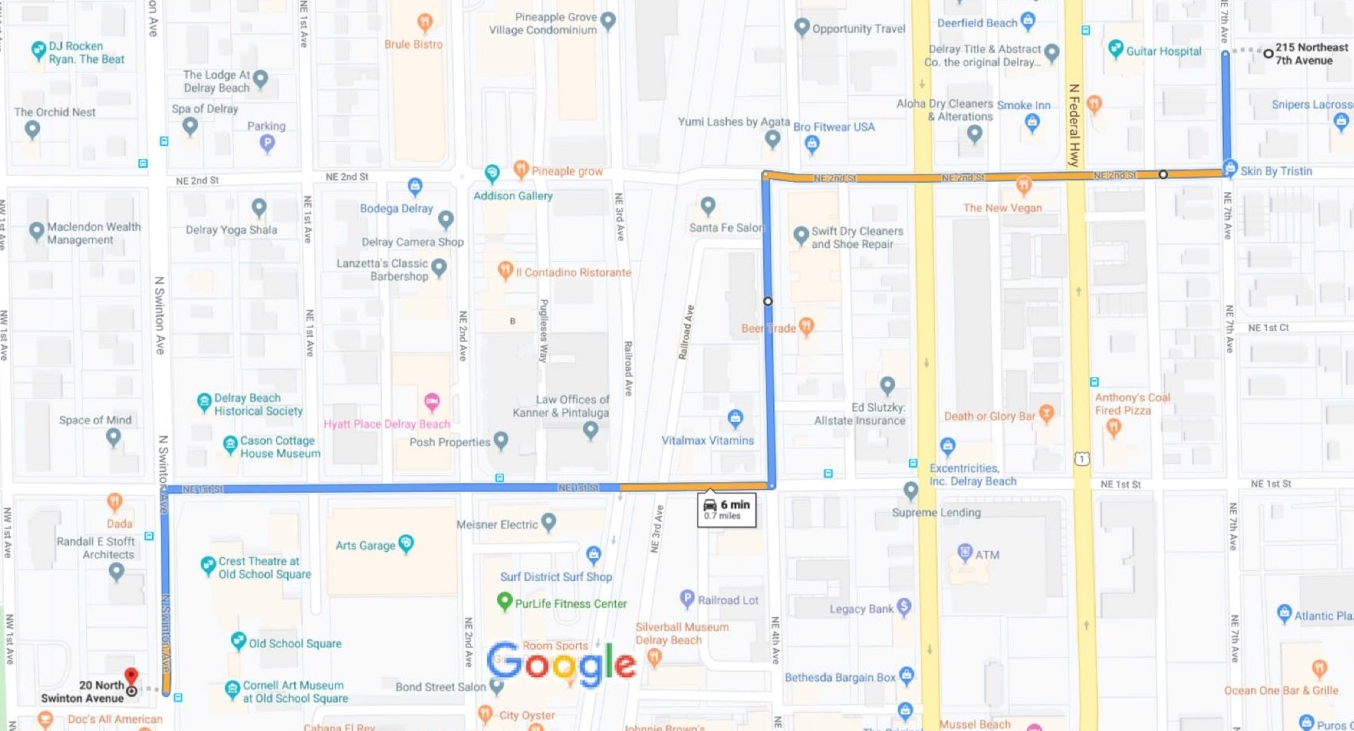Screenshot of a Google Maps navigation route within a bustling urban environment. The map is adorned with the familiar bright colors of the Google logo—blue, red, yellow, and green. The starting point is clearly marked at 20 North Swinton Avenue, positioned in the lower left corner of the display. The route plotted out by the user meanders north, then east, north again, followed by another eastward turn, and finally heading north one last time, culminating at 215 Northeast 7th Avenue. Along this intricate path, a variety of pins indicate numerous businesses, offering choices in dining, retail, fitness, and other amenities typical of a densely populated city. The map effectively highlights the vibrant commercial landscape of the area, promising an array of urban experiences.